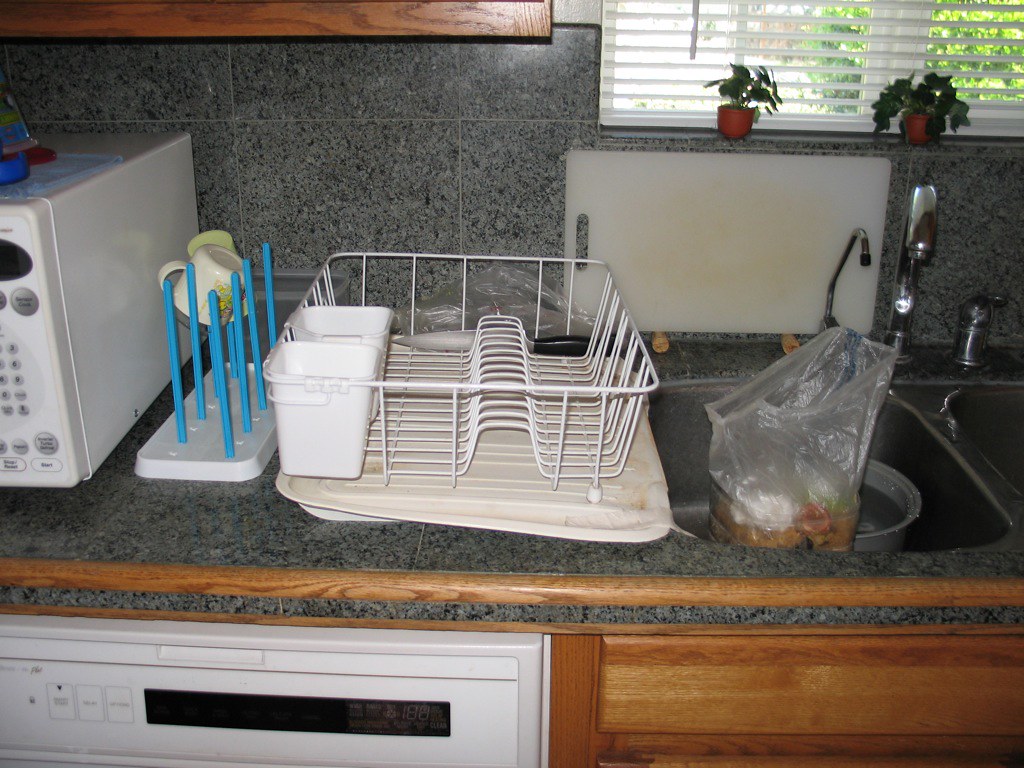This photograph captures a detailed scene of a busy kitchen countertop. To the bottom right of the frame, there is a reddish-brown wooden set of drawers. Directly to the left, a white dishwasher with a black digital screen displays faint white outlines of its output. The dishwasher features white buttons with gray text.

The countertop itself is a mottled gray stone with a contrasting wooden trim. On the left side, the right end of a deep white microwave is visible. The microwave is equipped with gray buttons and black text, as well as an oval black screen located at the top right.

Occupying the countertop is a small rack with a white base and blue stems designed to hold items for drying. Currently, the rack supports a beige mug and a lime green, possibly plastic, cup. Adjacent to the rack stands a white dish rack positioned on a white mat, designed to angle down towards the sink on the right. The dish rack features several upside-down U-shaped segments at its base and contains two white cups for utensils.

To the right lies the metallic sink, partially filled with a bag containing a variety of colored objects—white, red, orange, and green. Situated behind the bag is a gray dish filled with water. Leaning against the gray tile wall behind the sink is a white cutting board.

In the top right corner, a window adds natural light to the scene, flanked by two small plants with green leaves. Each plant rests in an orangish vase, injecting a touch of greenery and earth tones into the kitchen environment.